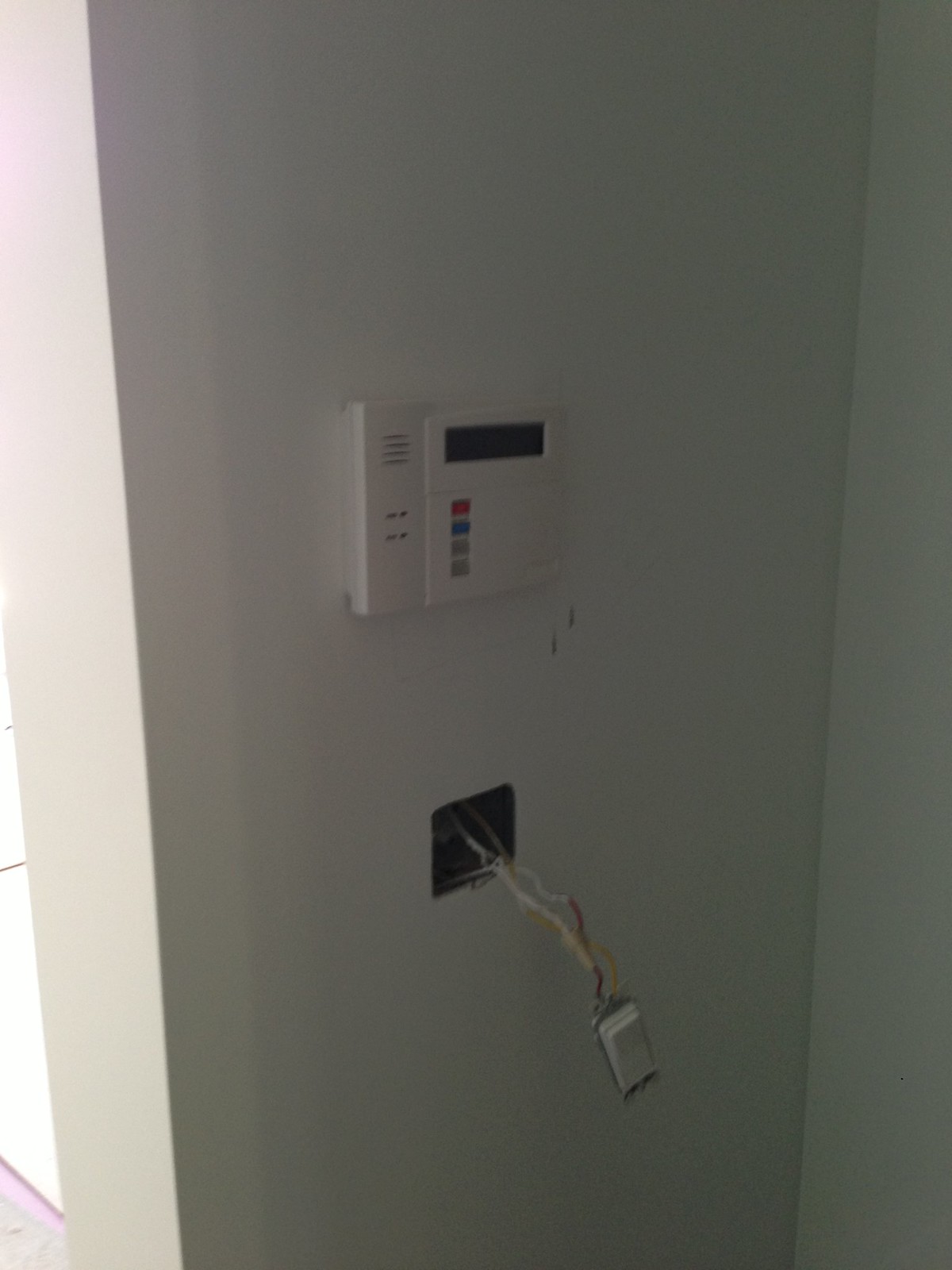This photograph captures the corner of a dimly-lit room, showcasing two intersecting white walls. The right wall is partially in shadow, adding a slightly darkened tone to the scene. Mounted on the left wall is a white plastic security system terminal featuring a rectangular gray screen at the top. Below the screen, there are four buttons in a vertical arrangement: the top button is red, the second button is blue, and the bottom two buttons are gray.

Further down the same wall, beneath the security terminal, there is a visible hole with some wiring protruding from it. Near the bottom of the wall, there is a flat white light switch. The left side of the photo hints at some light entering the room, possibly from a window, softly illuminating the scene.